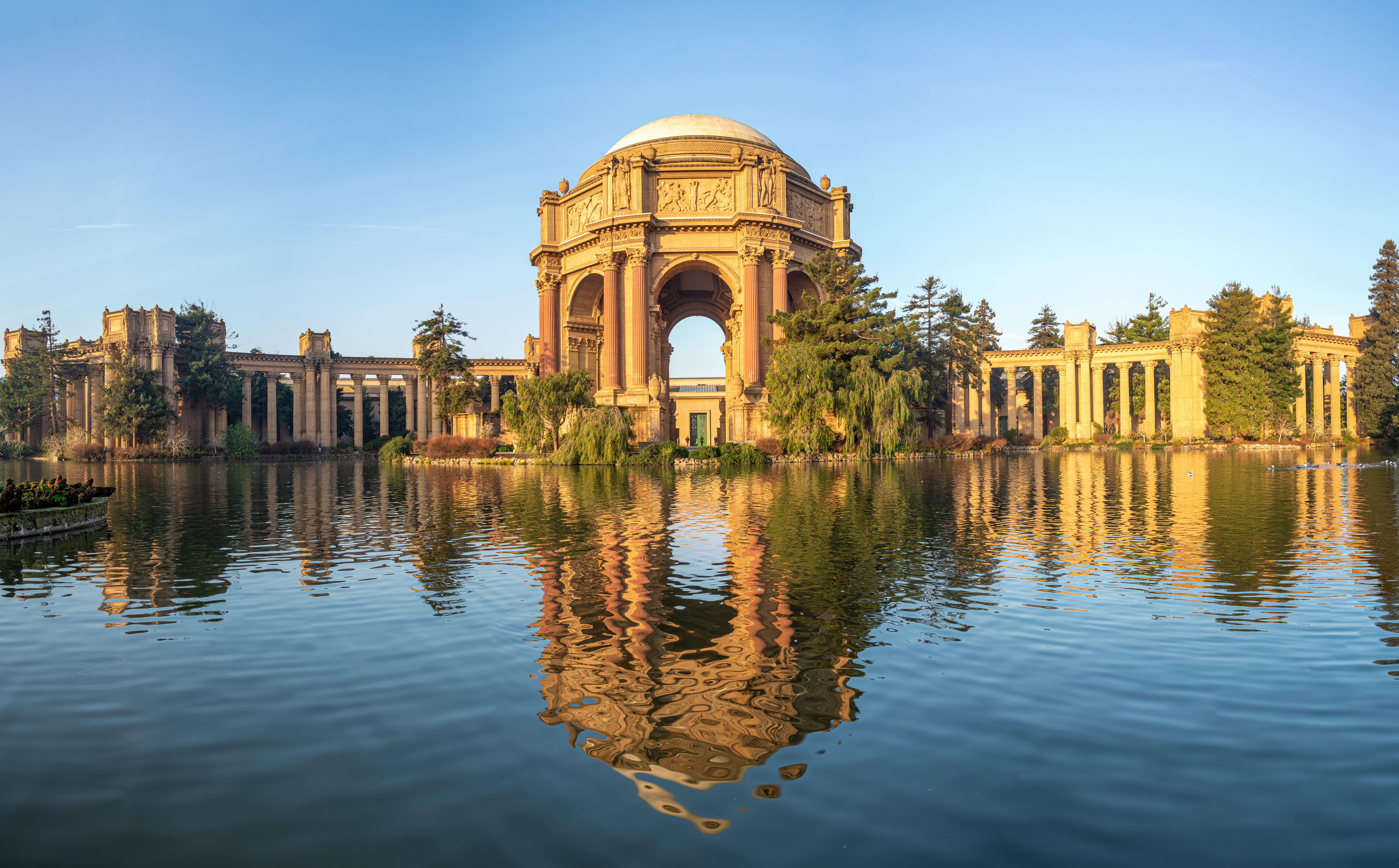The image features an exquisite building set against the serene backdrop of a calm body of water in the foreground. The structure, exuding an Indian architectural influence, is primarily constructed of sandstone-colored stone. At the heart of the building stands an open, domed structure with a striking white dome adorning its top. This central piece is characterized by a prominent keyhole archway that offers a glimpse of the smaller building behind it.

Flanking the central dome on both sides are symmetrical colonnades of Roman columns, each supporting a horizontal stone beam, all crafted from the same sandstone material. In front of the building, a small copse of trees adds a touch of natural greenery to the otherwise stone-dominated scene.

The building's elegant features are perfectly mirrored in the placid waters below, which appear to be a pond or lake. The setting is bathed in sunlight under a clear, bright blue sky, completing the picturesque and tranquil atmosphere.